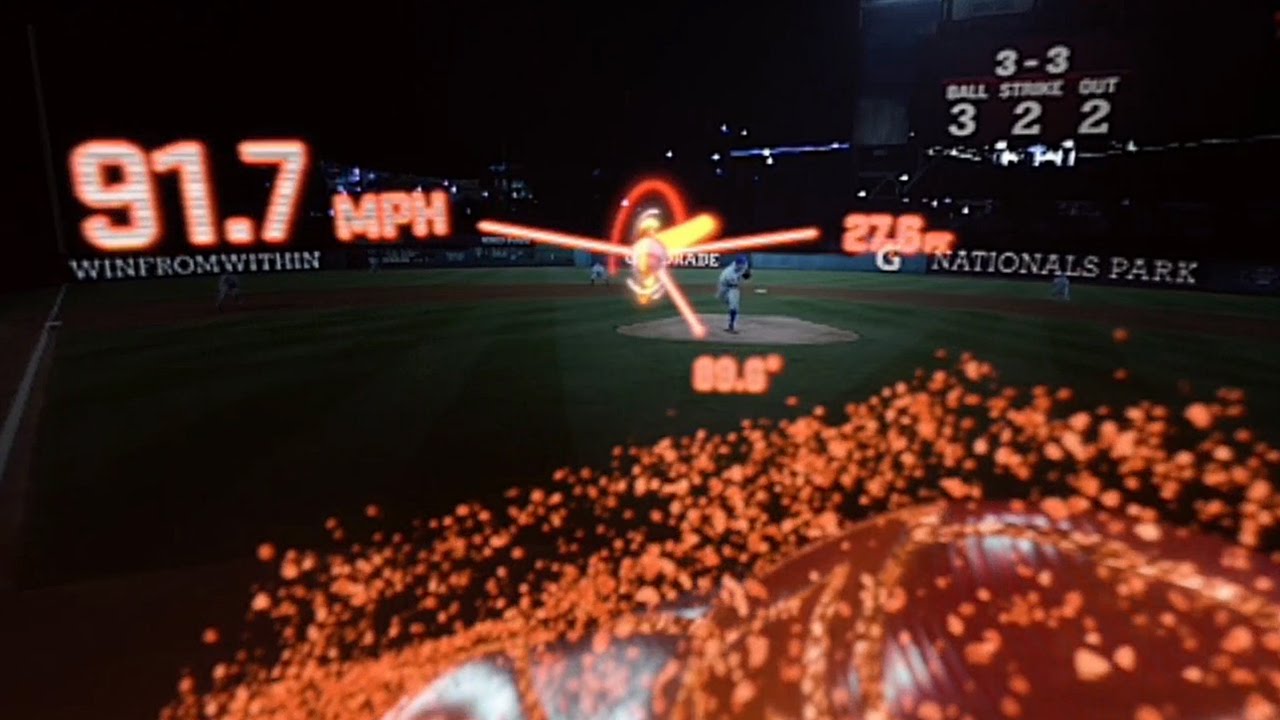The image depicts an intricate statistical analysis of a baseball game. At the center, a pitcher is captured in the act of throwing a fastball. Surrounding the fastball are several data points: its speed is marked at 91.7 miles per hour, the angle of the pitch is 89.6 degrees, and the distance covered by the ball is 27.6 feet. The background shows the baseball field with a green and brown ground, and players positioned across various bases including first, second, shortstop, and third.

A graphical element overlays the scene, featuring a ball in the center with glowing lines extending from it, each annotated with the previously mentioned statistical metrics. Additionally, the bottom portion of the image presents a close-up view of a red-colored ball surrounded by many orange dots.

In the top right corner, the scoreboard displays the game's standing, indicating a score of 3-3, with the current count being 3 balls, 2 strikes, and 2 outs. The scoreboard also notes "Nationals Park" and advertising banners in the outfield, including a Gatorade logo with the slogan "Win From Within." The stadium's seating area appears shadowy and dark, enhancing the focus on the analytics and the action unfolding on the field.